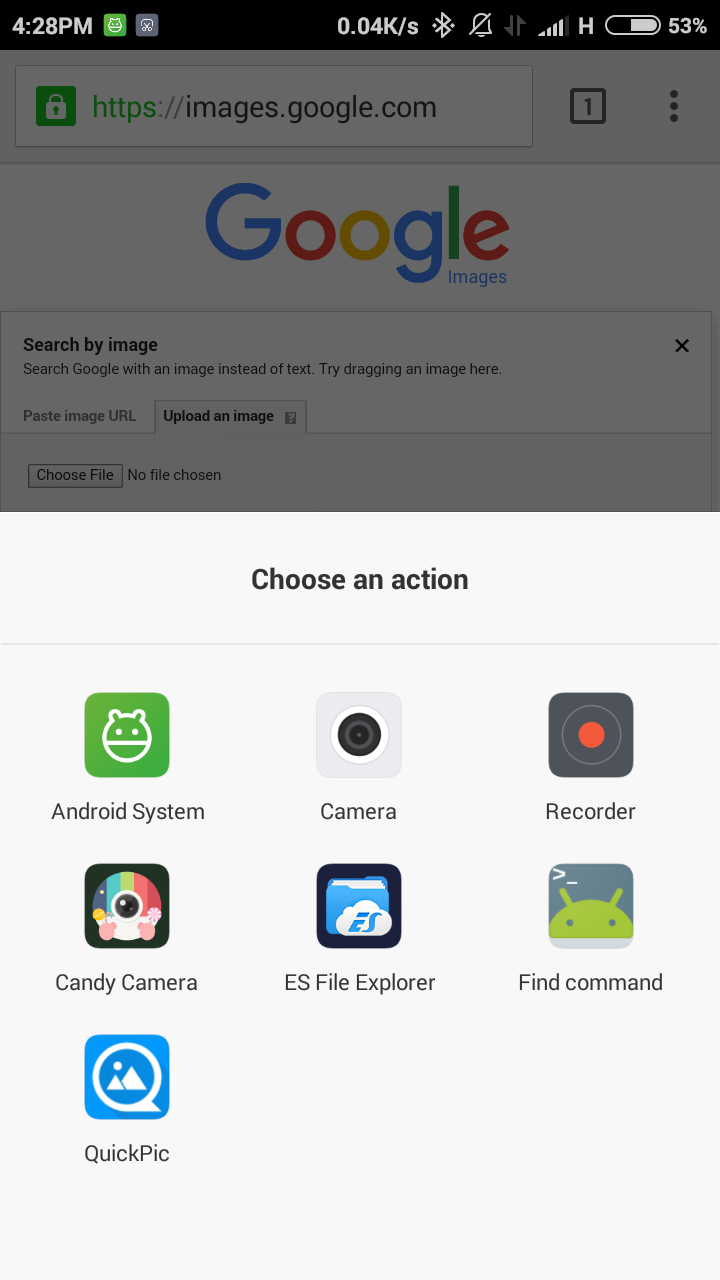This image displays a mobile device screen showcasing a website interface. Dominating the foreground is a semi-transparent overlay titled "Choose an Action," featuring multiple selectable links and icons. These options include:

- **Android System** icon
- **Camera** link
- **Recorder** link
- **Candy Camera** link featuring a colorful, rainbow-themed camera icon
- **ES File Explorer** link

Additionally, there are two buttons labeled "Find Command" and "Quick Pick."

The background reveals a slightly blurred view of the Google Images website at [https://images.google.com](https://images.google.com). This section includes the Google icon and text indicating options for searching by image rather than text: "Search by image, search Google with image instead of text." It prompts the user to drag an image to the designated area or to use the available options: "Paste image URL" and "Upload an image." At the bottom of the background section, there's a control labeled "Choose file," accompanied by the text "No file chosen."

The overall composition highlights a dual-layer view, with the darker, greyer overlay in the foreground that prompts the user to select an action and the Google Images interface subtly visible in the background, offering various image upload and search functionalities.